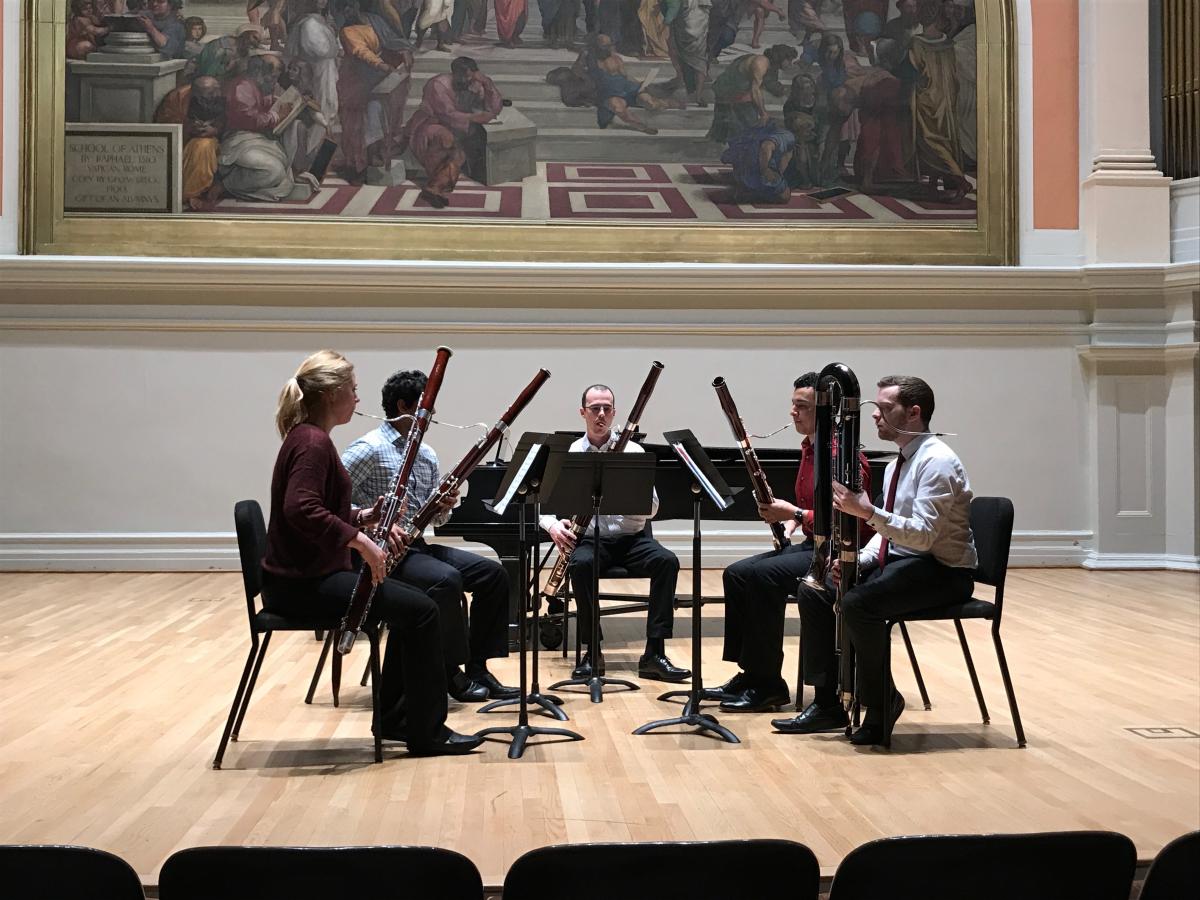In this detailed image, a small group of five oboists—comprising four men and one woman—are seated in a semicircle on a stage with a natural wood floor. The musicians, all dressed in black pants, are in the midst of a practice session, as evidenced by the absence of an audience and their focused attention on the sheet music before them. The woman, distinguishable by her blonde hair and burgundy shirt, contrasts with the men who are wearing a mix of white, blue, and burgundy shirts. Each musician has their own music stand and is seated on a black chair. Behind them, adding to the grandeur of the scene, is a large, ornate mural—possibly a reproduction of a famous painting from the Vatican by Raphael. The background also features some wood paneling and a black grand piano. In the foreground, the backs of empty fold-up chairs can be seen, indicating that the photograph was likely taken from the audience area of a very formal and classical-looking theater or museum space.